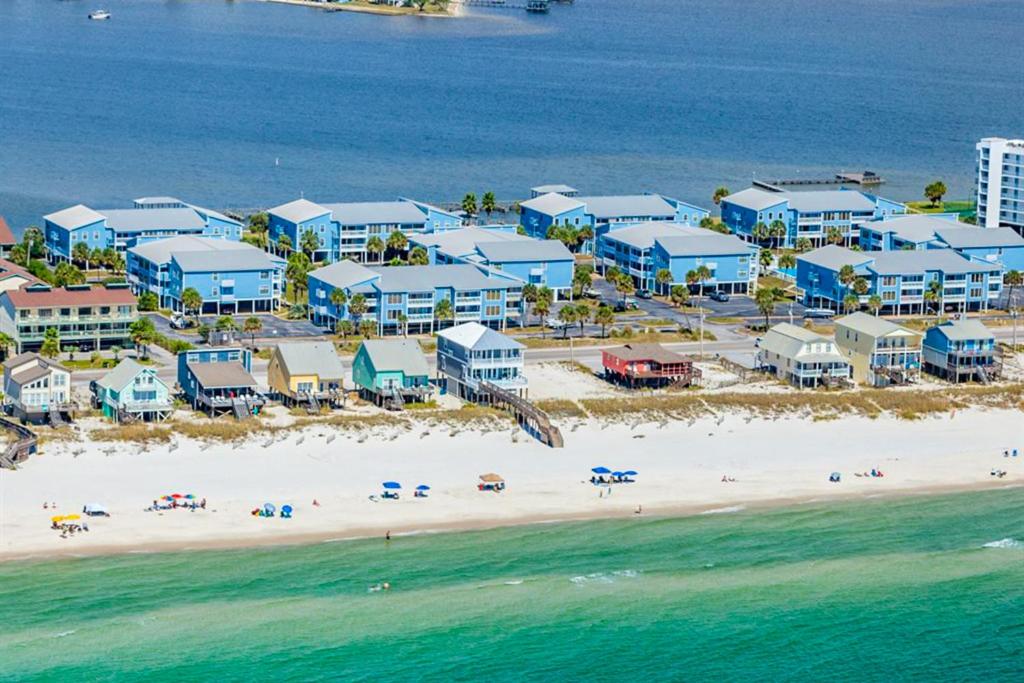The image depicts a narrow, heavily developed strip of land that appears to be either a small island or a spit reaching between two bodies of water. Along the edge of this strip, a broad white sand beach extends towards a lighter greenish-blue ocean, dotted with colorful umbrellas in blue, red, and yellow providing shade to a few beachgoers. A dune line fortified with plants stands behind the beach, leading to a series of beach houses, each elevated on stilts to mitigate flooding risks. One of these houses features a boardwalk staircase descending directly onto the sand, while the others have paths winding through the foliage.

Further inland, behind a road, stands a cluster of identical blue apartment buildings, also elevated on stilts, likely with parking areas beneath them. These apartments are organized in two or three neat rows, creating the impression of a planned development. The strip's top side features a darker blue section of the ocean, contrasting with the lighter hues of the water below. The landscape shows a gradient from beach to residential areas, capped by the vast, differing expanses of the sea, hinting at a transition from a greener, more shallow area to deeper waters. In the distance, another tiny island is visible alongside a small boat near the top left corner.